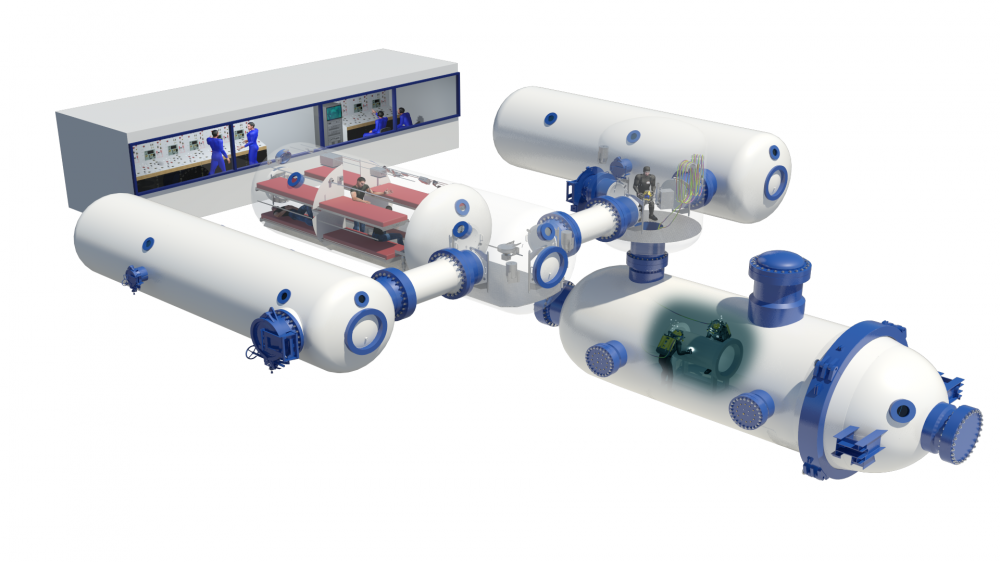The image is a highly detailed 3D illustration of an underwater habitat or base, showcasing various interconnected cylinders and tubes, likely used for scientific or military experiments. Large white tubes, connected by blue pipes and secured with riveted mounting points, form the structural framework. These tubes serve different functions, including living quarters and specialized chambers, seamlessly linked by smaller passage tubes.

In the center, a prominent canister features multiple bunk beds and houses several human figures in blue uniforms, suggesting a living or resting area. Adjacent to this central chamber, two other transparent chambers reveal intricate activities: one depicting a man in a wetsuit, and the other showing two individuals fully equipped with scuba gear, indicating underwater or pressurized environment training.

The habitat includes a control center on the far left, distinguishable by its large windows and numerous control panels. Inside, more individuals in blue uniforms manage and monitor operations, likely evaluating data from their computer screens. Additionally, in one of the cylinders, a man can be seen immersed in water, further emphasizing the facility's function as an experimental or training environment for underwater activities.